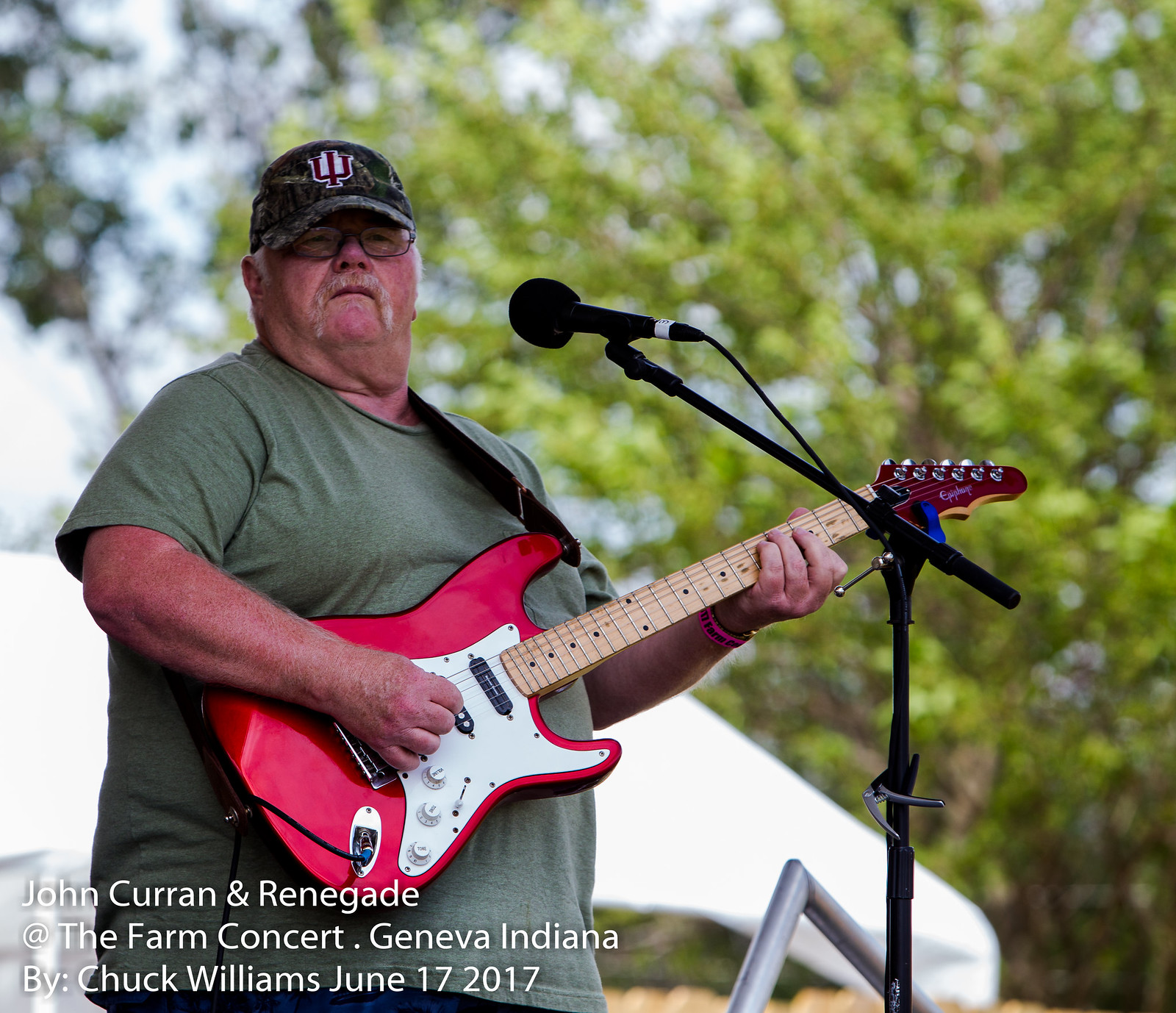In the image, we see a man on an outdoor stage, playing a red and white guitar, with a microphone positioned right in front of him. He is wearing a camouflage baseball hat with a trident logo, glasses, and a green t-shirt. He sports a distinct long, white mustache. The environment around him suggests he is at a live event, given the white tent behind him and the blurry trees with green leaves that form the background. The sky peeks through in a blurry bluish hue. In front of him, there is a triangular-shaped armrest or guardrail. At the bottom left of the image, text reads: "John Curran and Renegade at the Farm Concert, Geneva, Indiana, by Chuck Williams, June 17, 2017."